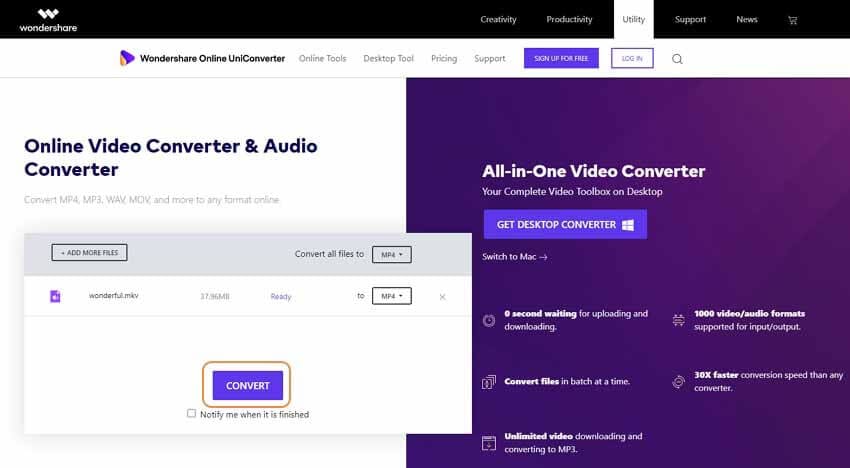A horizontal-oriented screenshot of the Wondershare website is displayed. The name "Wondershare" is prominently featured in the upper left-hand corner on a black banner, accompanied by a white "W" logo. To the right, there are drop-down menus labeled as Creativity, Productivity, Utility (highlighted in white), Support, and News, along with a shopping cart icon. 

Below this black banner, another white toolbar shows "Wondershare Online Unit Converter" on the left, followed by options for Online Tools, Desktop Tool, Pricing, and Support. Towards the right end of this toolbar, there is a purple "Sign Up for Free" button, a Login button, and a magnifying glass search icon.

The webpage's main section features a white background on the left and a dark purple background on the right. Overlapping these backgrounds is a pop-up white text box with a large purple "Convert" button. On the left section of the main area, the text "Online Video Converter and Audio Converter" is visible. The right section reads "All-in-One Video Converter" with a "Get Desktop Converter" purple button. Below this, several icons signify features such as "Second, Waiting for Uploading and Downloading," "Convert Files in Batch at a Time," "Unlimited Video Downloading and Converting to MP3," "1,000 Video/Audio Formats," and "30 Times Faster."

In the left pop-up box, there are options for "Add More Files" and a drop-down menu labeled "Converting Files to." Beneath the purple Convert button, there is a checkbox labeled "Notify Me when it is finished."

Overall, this comprehensive screenshot provides a detailed view of the Wondershare website's various tools and navigation components, highlighting the online video and audio conversion features.